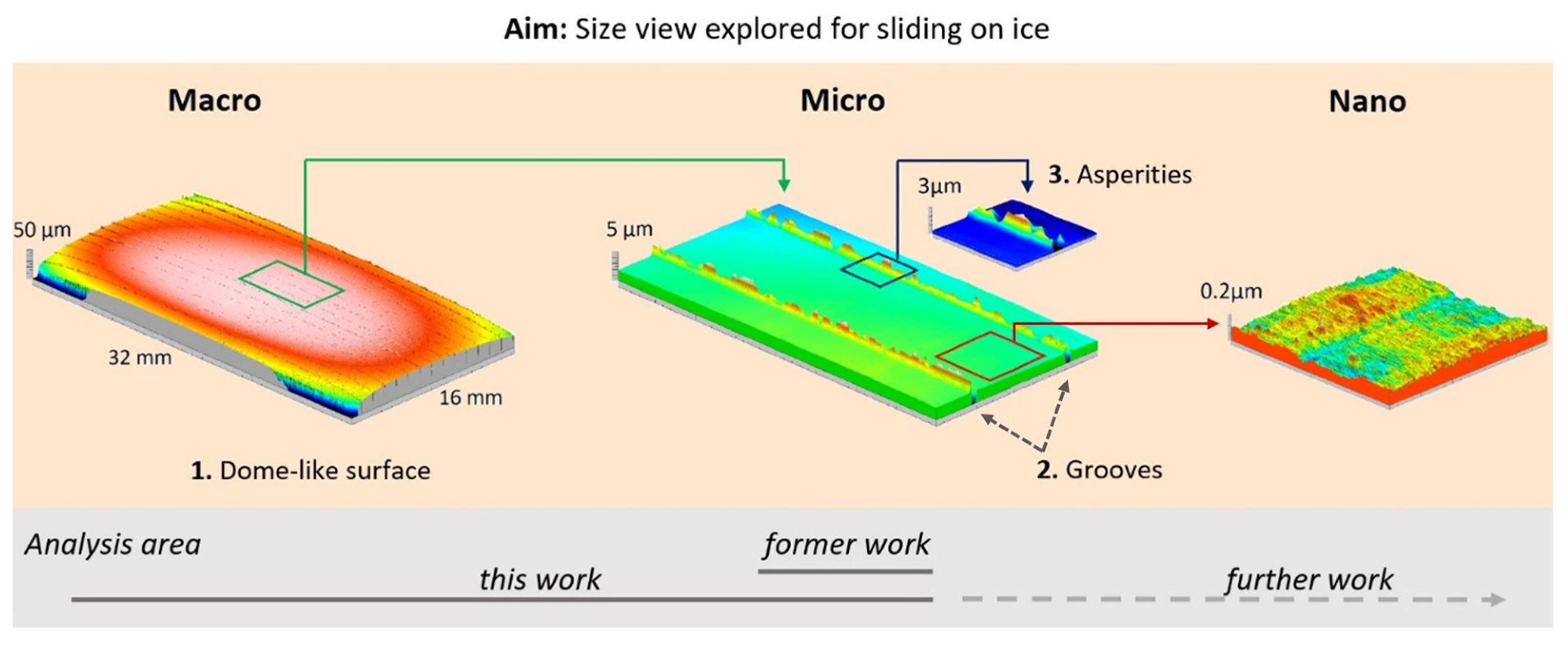The image is a detailed scientific diagram from a textbook, showcasing the exploration of surface structures for sliding on ice. The title at the top in bold reads "AIM," followed by "Size view explored for sliding on ice" in regular font. The diagram is presented in a landscape layout and features three sections labeled according to scale: macro, micro, and nano. Each section has its own distinct diagram depicting surface appearances in vibrant colors ranging from red, yellow, green, to blue.

In the macro view, measuring 32 millimeters by 16 millimeters, there's a heat map with a red dome-like surface transitioning through yellow and green to blue, representing the "dome-like surface." The micro view mainly shows green with yellow bands and some details marked as "grooves" and "asperities." The nano view displays ridges of yellow and green.

Beneath the diagrams, a line indicates an "analysis area," which progresses from "this work" to "former work" and "further work," providing a timeline for the research conducted. The overall illustration appears to be a computer-generated scientific representation highlighting differences in surface structures across varying scales.